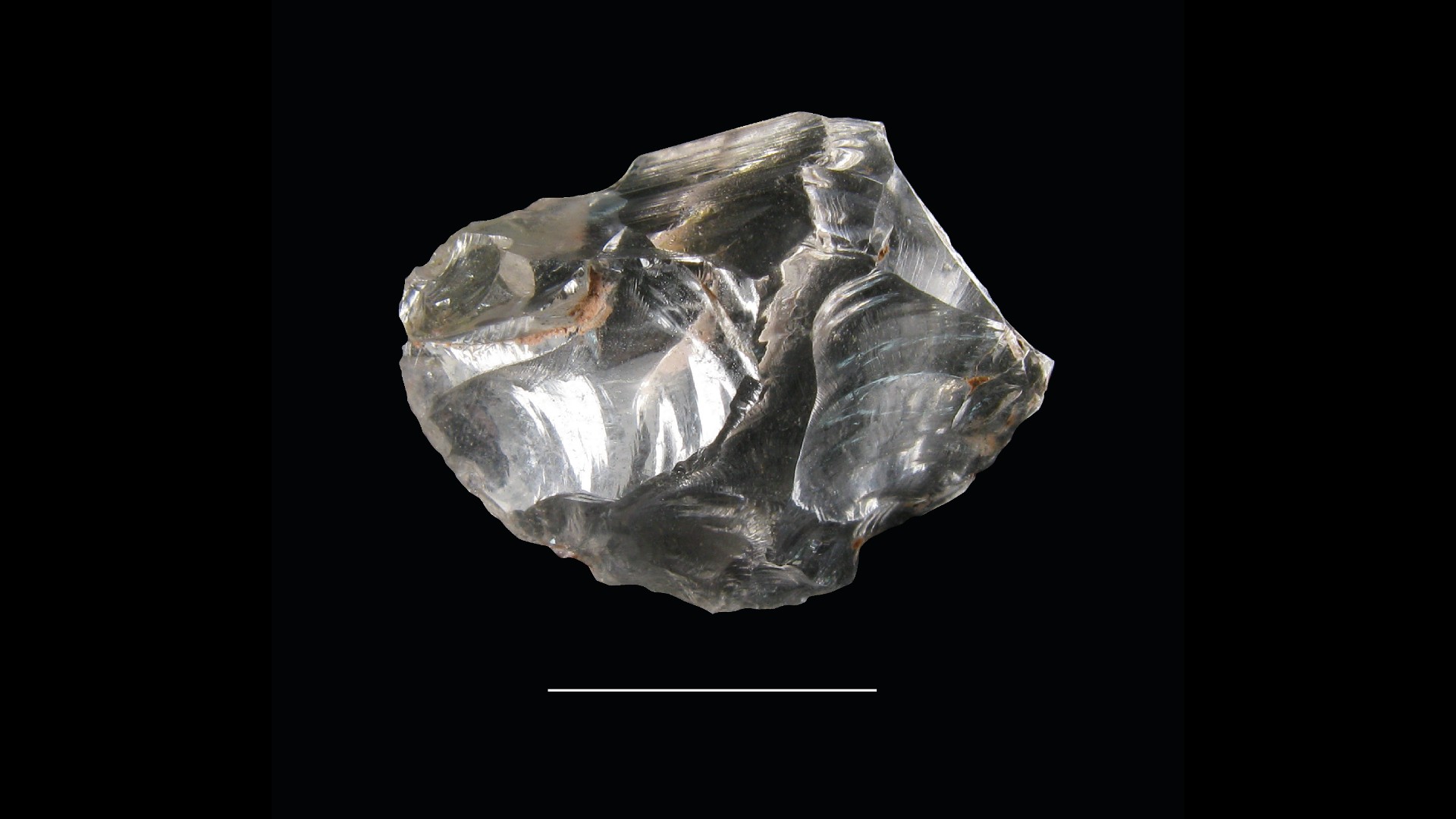This rectangular image measures approximately 6 inches wide and 3 inches high and features a predominantly black background with darker vertical borders, around an inch wide, on both the left and right sides. The central area of the background is a slightly lighter grayish black. In the heart of the composition lies a rough, uncut gemstone or possibly a piece of milky white translucent quartz. The gem exhibits several prominent curved fractures and blemishes with orangish dirt specks visible on the upper left and central right areas. The ridges and texture of the gem catch and reflect light, particularly on the left side, adding to its intricate and unpolished appearance. Below the gemstone, a thin, 1-inch horizontal white pinstripe spans across the bottom of the image, anchoring the composition.